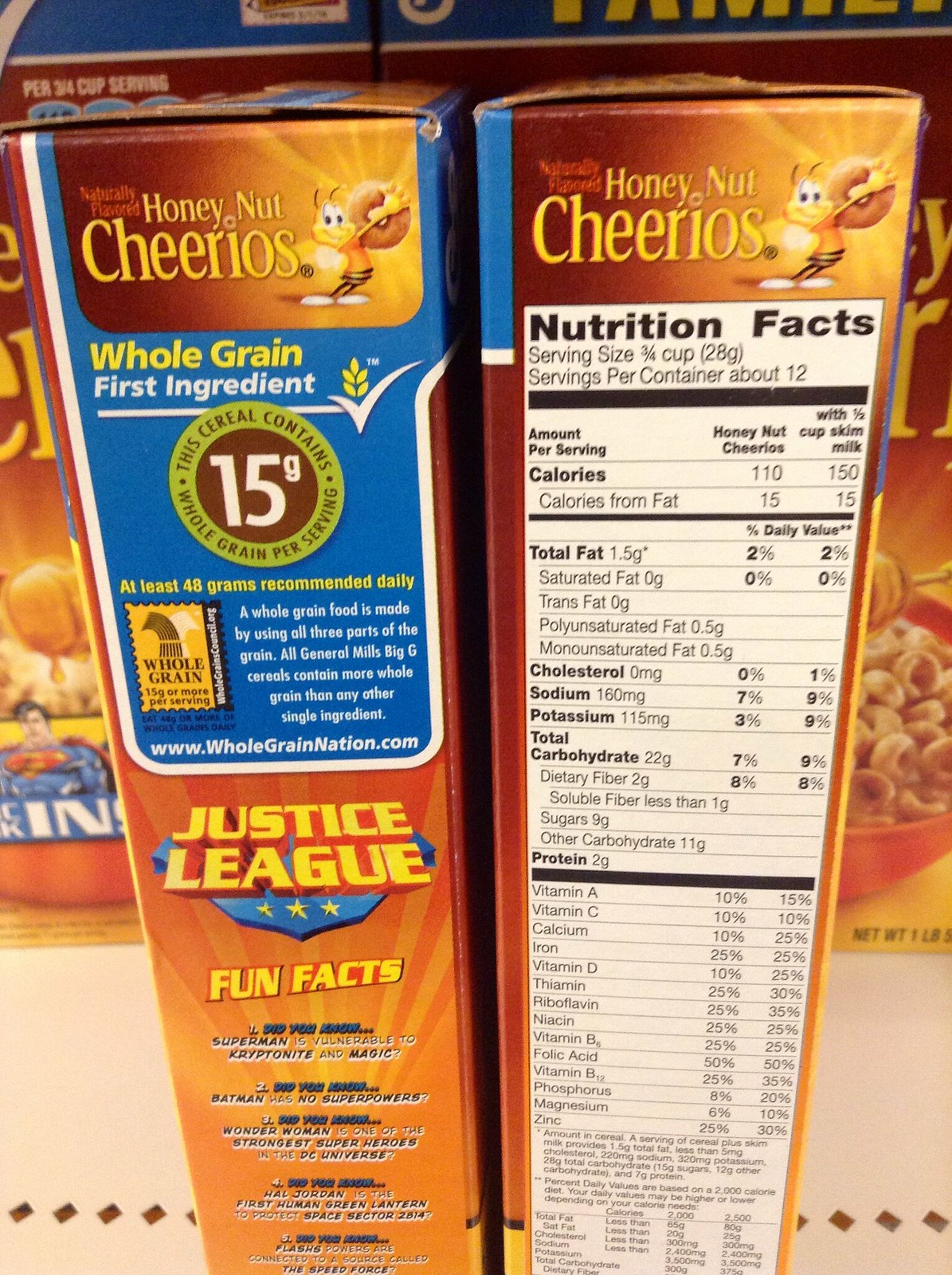This image showcases a variety of cereal boxes, with a particular focus on two prominently displayed Honey Nut Cheerios boxes oriented sideways. The engaging composition allows a detailed view of both sides of these boxes. They exhibit a rich, gradient color scheme transitioning from deep oranges to lighter yellows, encapsulating a vibrant honey-golden tone. A small, animated yellow honeybee donning black and yellow stripes is featured on the boxes, holding a golden piece of cereal above the prominent "Honey Nut Cheerios" label in bold yellow letters.

The box on the right side prominently features detailed nutrition information presented within a light-colored box with dark, easy-to-read letters. In contrast, the left box highlights the cereal's health benefits with a blue section that states, "Whole grain, first ingredient," and notes that each serving contains 15 grams of whole grain. Further enriching the visual and educational appeal, the bottom section of these boxes includes "Justice League" fun facts, offering an engaging read for the viewer.

In the background, additional cereal boxes are visible, although mostly obscured by the tight framing on the two main Honey Nut Cheerios boxes, suggesting a larger collection just out of view. The arrangement and detailed depiction of the cereal boxes provide a vibrant and informative snapshot of breakfast options.